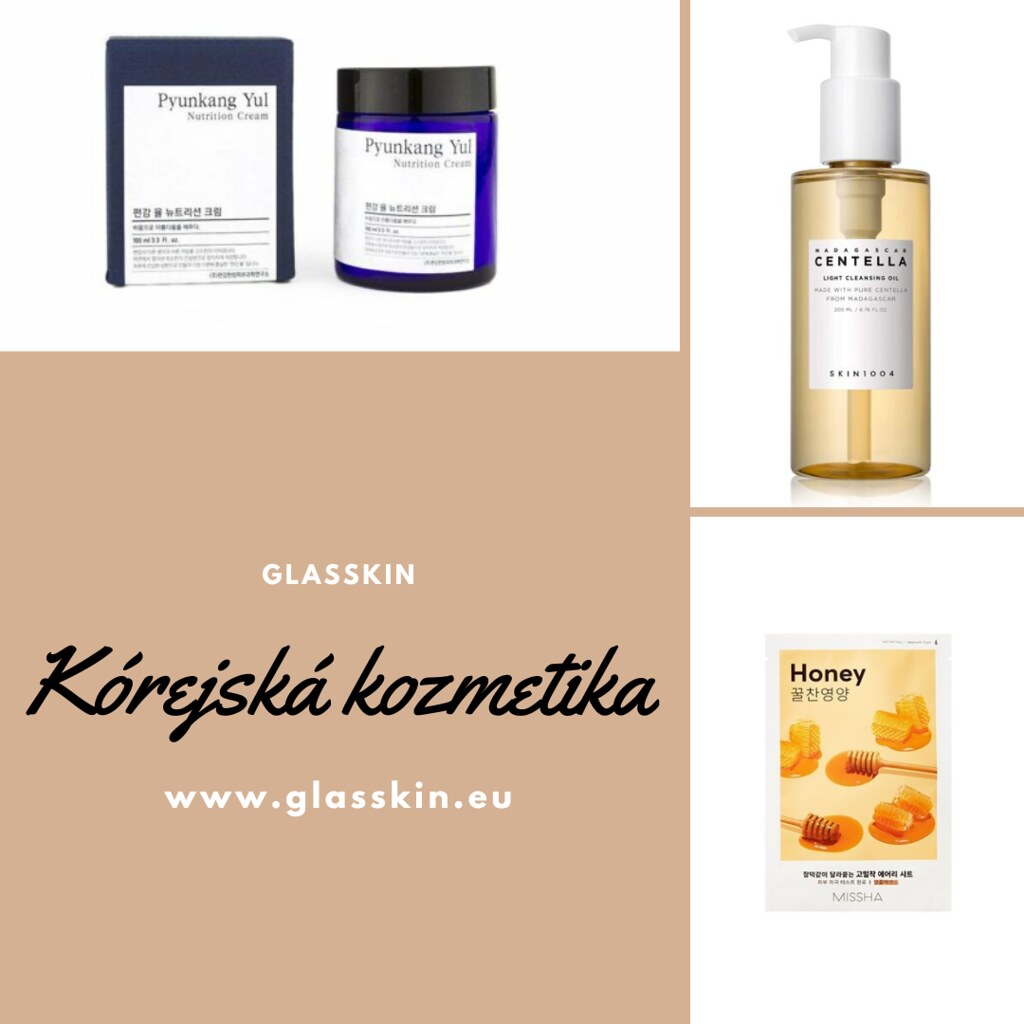This advertisement for www.glasskin.eu showcases various beauty products meticulously arranged in four distinct boxes. In the upper left-hand box, there is a product labeled "Punyuk Yun," which seems to be a hand cream or medicinal item, presented in a blue jar with a black lid. The upper right-hand box features a foaming cosmetic product in a tan pump bottle labeled "Centella," containing a clear liquid. The lower right-hand box highlights a product related to honey, depicting honeycomb pieces immersed in pools of honey alongside a honey dipper. The lower left-hand box contains the name of the brand, "Glass Skin," the website URL, and a foreign phrase including the word "Cosmetica." The color palette of the advertisement includes shades of blue, black, tan, orange, and the rich golden hues of honey.